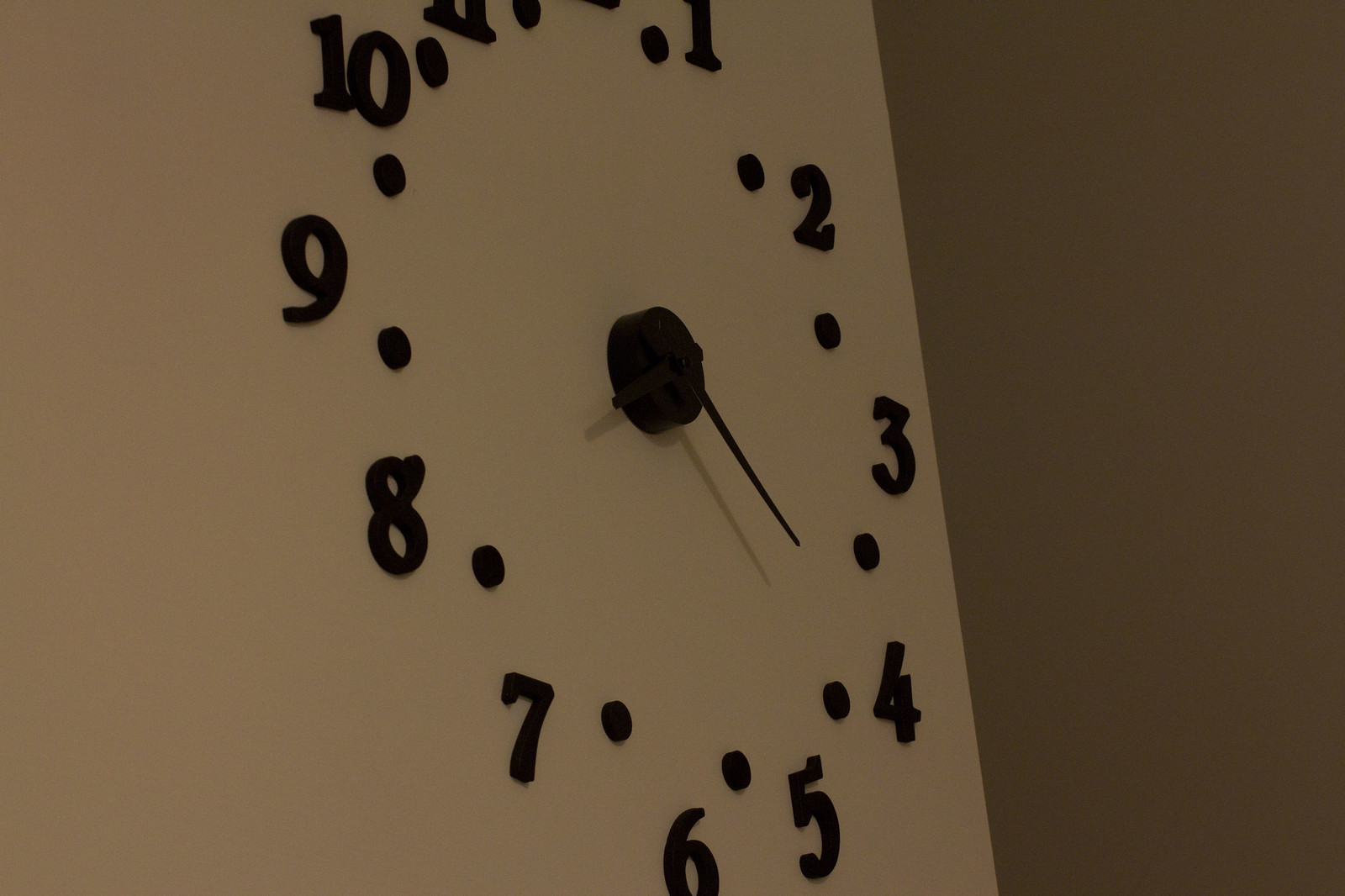The image showcases a minimalist wall clock directly mounted on a wall, positioned at an angle that reveals both the left and right sides of the room. The right wall is painted a rich brown, while the left wall boasts a very light taupe hue. The clock itself is frameless, consisting of numbers 1 through 12 individually adhered to the wall, each separated by small dots that likely indicate the half-hour marks. The clock hands are anchored by a central piece resembling a hockey puck, also attached to the wall. The current time displayed on the clock is 8:20. The overall aesthetic is simple yet modern, and the photograph is taken from a slightly off-center perspective, adding depth and dimension to the composition.